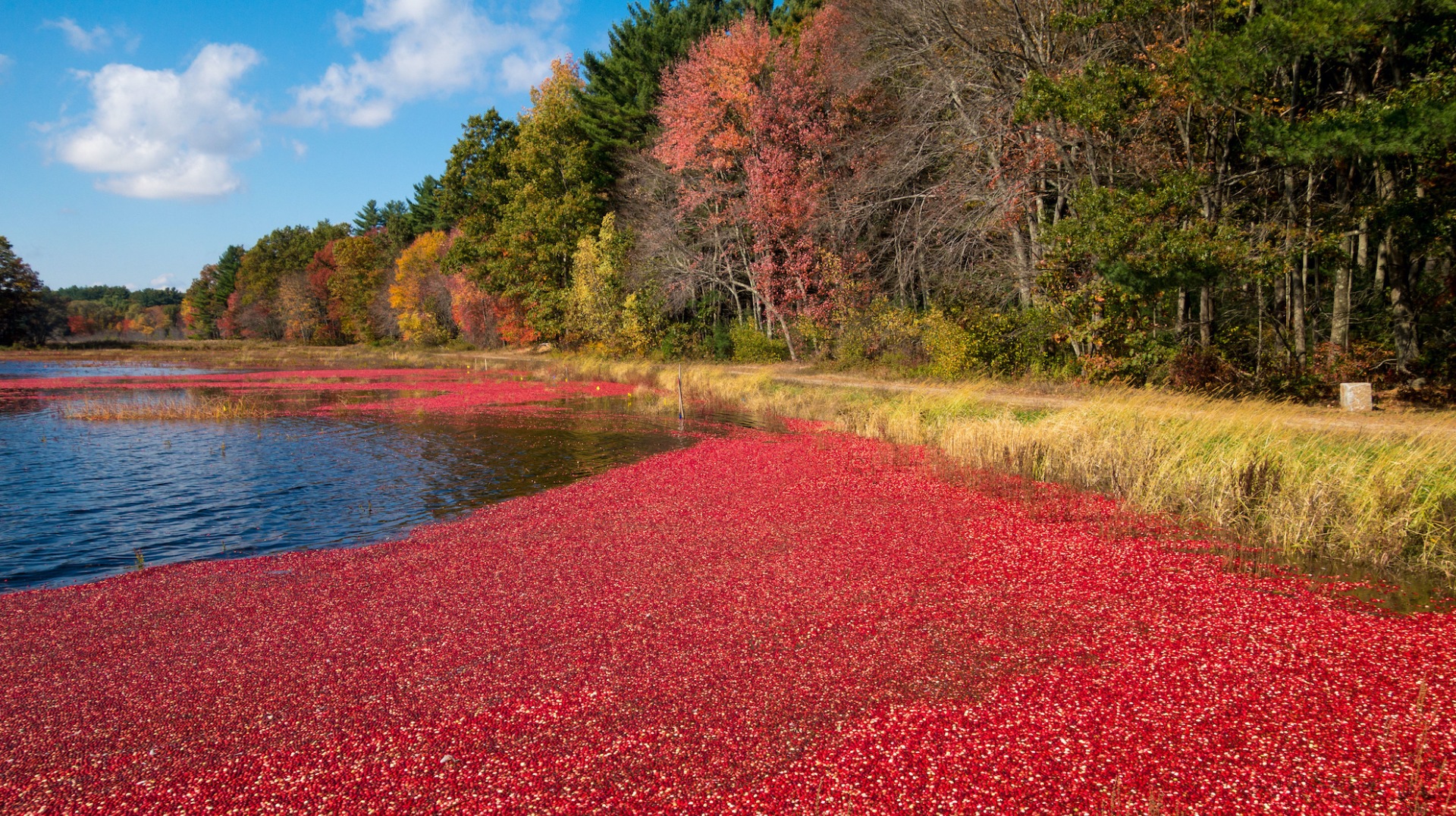The image depicts a serene autumn pond, partially covered with floating red cranberry plants, creating a vivid contrast against the dark green and deep blue hues of the remaining open water. The pond is bordered by tall grasses and a narrow dirt road that runs parallel to its edge. Beyond the road, a densely wooded area features a mix of evergreens and deciduous trees, their foliage transitioning into vibrant shades of yellow, orange, and red, emphasizing the season. The sky in the top left corner is a bright blue, dotted with a few white clouds, adding to the tranquil and picturesque scene. The abundance of red cranberries floating on the water's surface in the foreground highlights the unique and surreal beauty of this autumnal landscape.